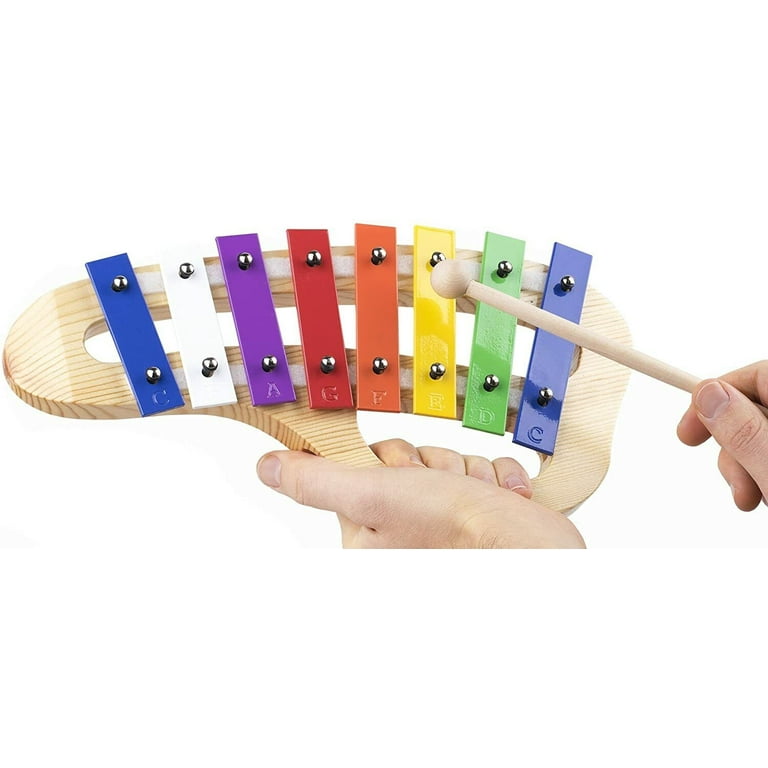The image shows a person engaging with a colorful xylophone, centrally positioned in a bright, white backdrop. The xylophone features vibrant bars in hues of blue, white, purple, red, orange, yellow, and green, along with a wooden base in beige shades. The bars are distinctly labeled with letters—'A' on the purple, 'F' on the orange, 'D' on the green, and 'C' on the blue—suggesting an educational, child-friendly instrument. The person's hands, appearing from the bottom middle and bottom right of the image, grasp the xylophone and a mallet, respectively, poised to produce music.